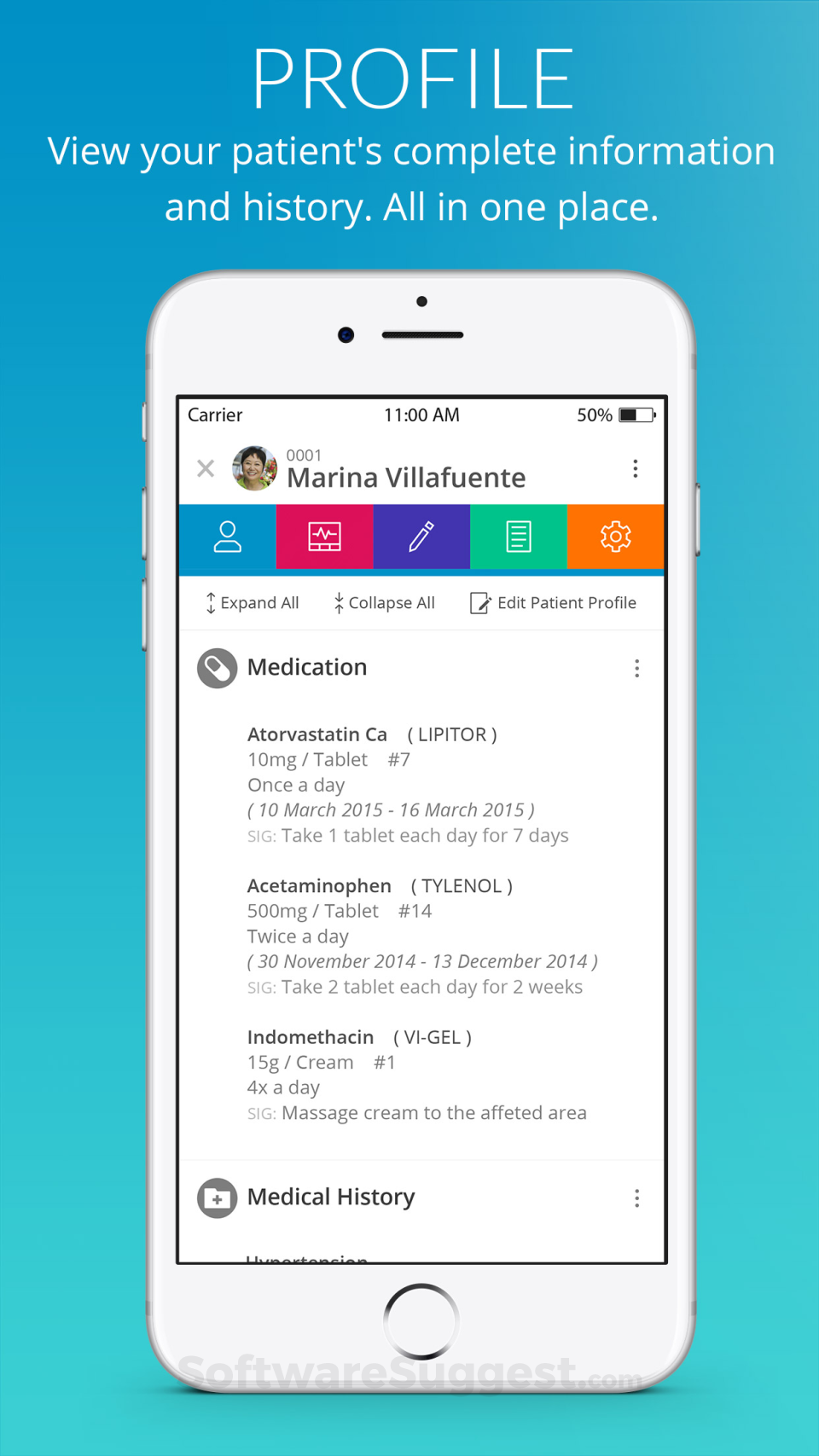The image features a background with an ombré gradient in aquamarine. Overlaying this background, the phrase "Flag as inappropriate" is displayed prominently. At the top of the image, "Profile" is written in white, and beneath it, in all capital letters, are the words: "VIEW YOUR PATIENT'S COMPLETE INFORMATION, EXCELLENT, AND HISTORY. ALL IN ONE PLACE."

In the foreground, there is a white iPhone. The screen of the iPhone has a white background displaying various details. At the top of the screen, the word "Carrier" is visible in black, along with the time "11:00 AM" and a battery icon indicating 50% charge. 

On the screen, several names, including "Marina Filafute," are listed, each accompanied by several icons: 
- A blue square with a person icon
- A red square with an icon resembling a box with zigzag lines
- A purple square with a pen icon
- A green square with a piece of paper icon
- An orange square with a gear icon 

Below these icons, the section titled "Medication" lists various medications: 
1. Atorvastatin, to be taken once a day 
2. Acetaminophen (misspelled as "A-C-T-A-M-I-N-O-P-H-E-N"), to be taken twice a day 
3. Indomethacin (misspelled as "I-N-D-O-M-E-T-H-A-C-I-N"), to be taken four times a day